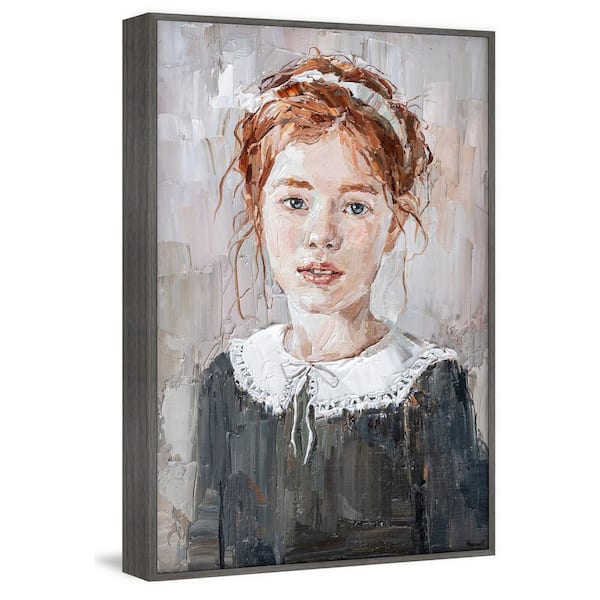The painting depicts a young, red-haired girl rendered in a large, close-up format. She gazes slightly to the side with her striking blue eyes partially hidden by her straggly red eyebrows. Her lips, naturally reddish-brown, are slightly parted, revealing her two front teeth. The girl wears a white hairband and a distinct white collar that wraps around her neck, resembling a doily. This collar, adorned with intricate embroidery around its perimeter, ties neatly at her chest over a dark, shaded-gray dress, typical of a protestant uniform. The canvas features a background blended in neutral tones of gray, pink, and white, adding a subtle elegance. The painting is framed with a thin gray border, highlighting the delicate, artistic composition of the piece.